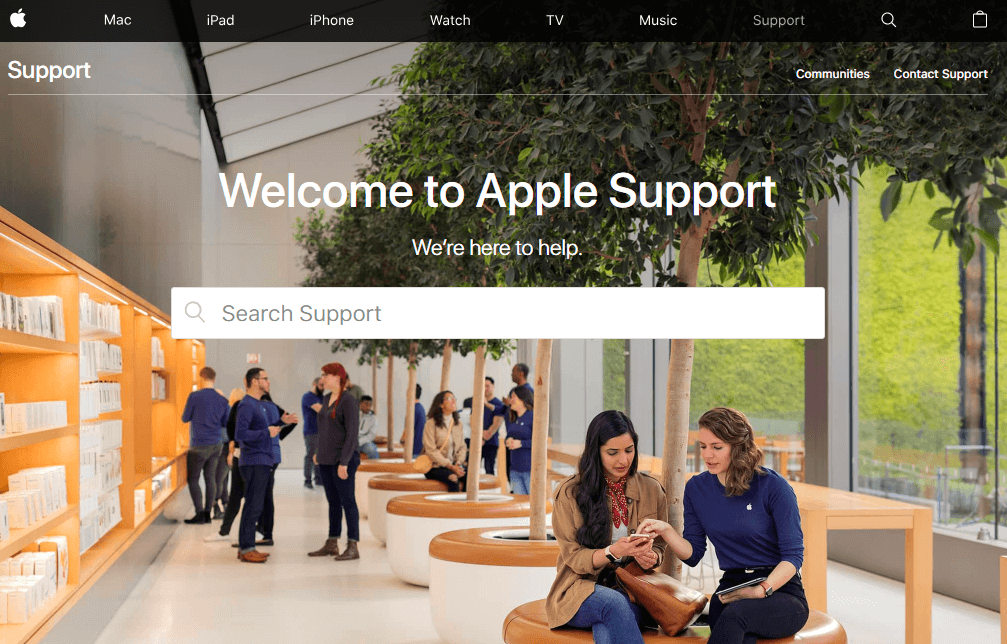This is a detailed screenshot of a webpage from a corporate website. At the top of the page, there is a black header featuring a white logo of an apple with a distinguishing curved bite taken out of its right side. Following this logo, there are labels spaced out horizontally in white text, reading: "Mac", "iPad", "iPhone", "Watch", "TV", and "Music". Further along, the word "Support" appears in light gray. Moving to the far right, there is a white magnifying glass icon for search functionality, followed by a white clipboard icon.

Below the header lies the main content of the page. The background consists of a photograph depicting a corporate office space. Large windows on the right side showcase a vibrant green wall of ivy. To the left, orange wooden shelves display white boxed products. Planters with wooden tops and white bases are positioned to the left and around the area, some of which have people sitting on them, with two individuals prominently in the foreground and several more in the background. Additionally, people are seen standing on a white floor to the left of the shelves.

In the top-left corner of the photo, there is white text that reads "Support". On the top right of the image, smaller white text says "Communities" and "Contact Support". Beneath this section is a thin white dividing line. Centered at the top of the next section is a large white text that says "Welcome to Apple Support". Below this, a line of smaller white text reads "We're here to help." Finally, a white search bar is situated underneath these lines of text.